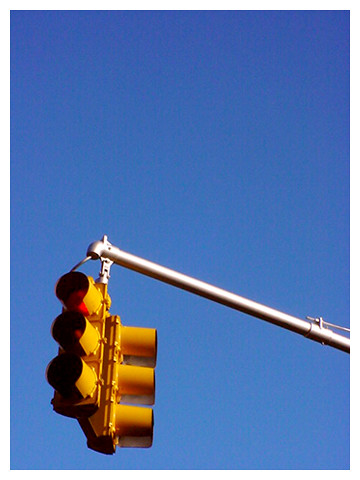This photograph captures a vivid street scene under a flawless, cloudless sky painted in a perfect sky blue. Dominating the image is a stainless steel metal pole extending from the right to the left of the picture, catching the sunlight on its shiny right side while remaining shaded on the left. Suspended from this pole is a bright, dark yellow traffic signal housing two sets of vertical lights. Each set consists of three bulbs arranged sequentially with red on top, yellow (amber) in the middle, and green at the bottom. The signal facing the camera glows red, suggesting that the lights on the opposite side are likely green. The traffic lights are angled upwards and to the left, creating a dynamic perspective in the photograph. The intricate details of the traffic signal's construction are visible, including the connecting edges and parts of the metal pole, making it a striking image of urban infrastructure against the serene blue sky.